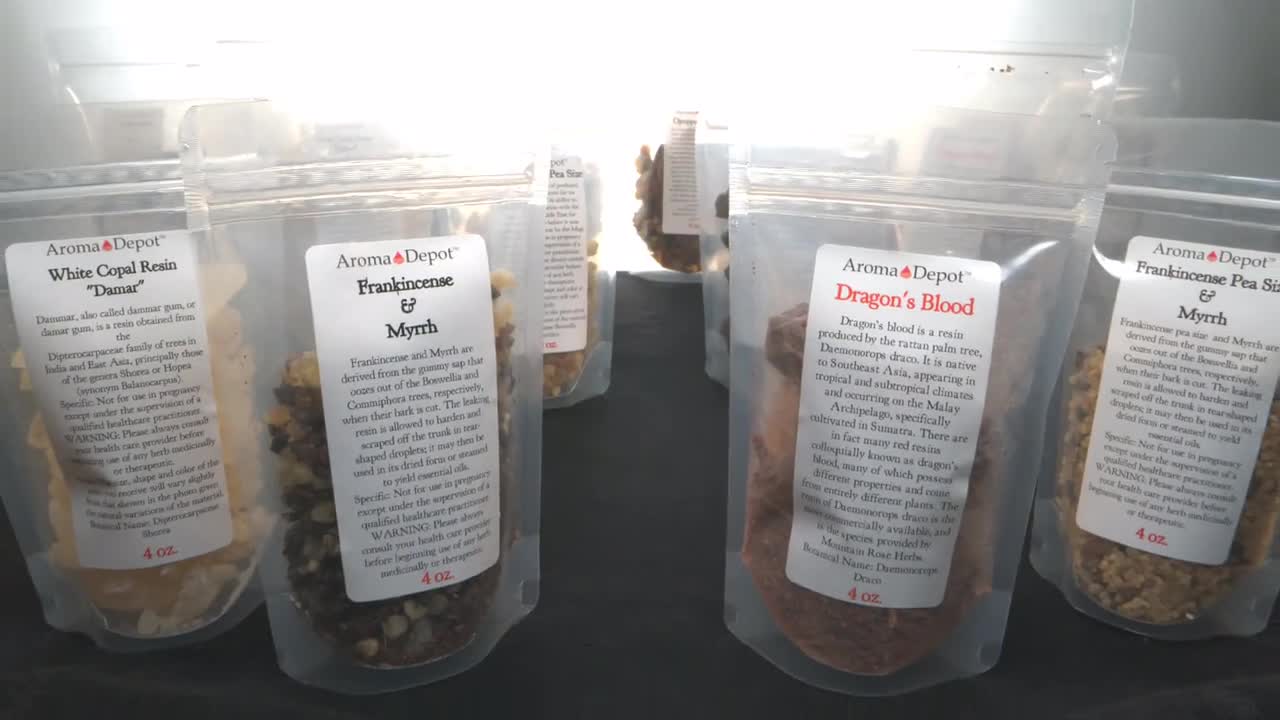The photograph is a horizontally aligned rectangular image featuring resealable, transparent plastic bags standing upright. The top part of the picture is slightly blurry due to the sunlight shining through a window. Each bag displays a vertical white label with the Aroma Depot logo printed in small black text at the top center. The type of aroma contained is listed beneath the logo: from left to right, the bags are labeled "White Copal Resin Damar," "Frankincense & Myrrh," "Dragon's Blood" (with the text in red), and an incomplete "Frankincense P6 & Myrrh," as the word is partially cut off. All the bags are four ounces, as indicated in red text at the bottom of each label. Detailed paragraphs about the contents appear beneath the aroma names. Behind and around these primary bags are additional similar bags, suggesting a variety of products intended for uses such as diffusers, incense, candle making, soap making, and body use.